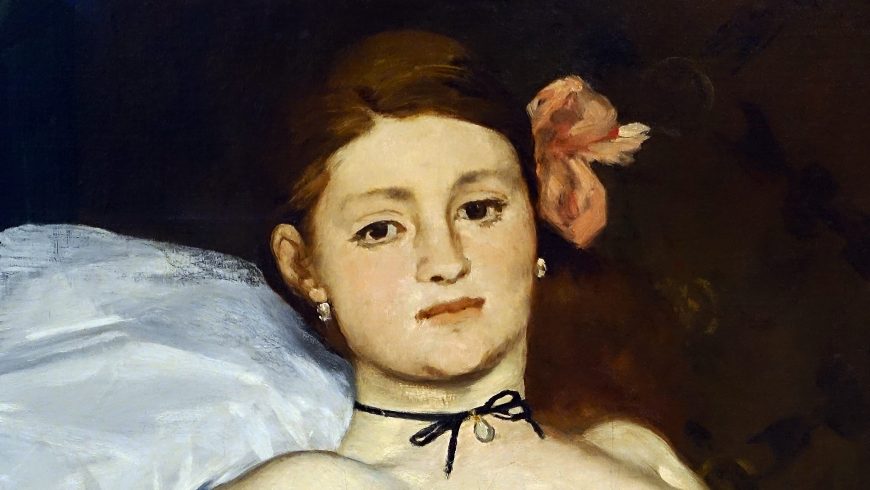This is an elaborate 19th-century oil painting featuring a young Caucasian woman, likely in her 20s or 30s, with intricate, heavy brush strokes reminiscent of the impressionist style or perhaps Toulouse-Lautrec. The woman has auburn hair styled back, adorned with a peach-colored flower tucked behind her right ear. She is wearing small, dangling silver earrings and a black choker tied in a bow, from which a jewel dangles. The woman is depicted reclining on a white, pillow-like surface, and she is staring directly ahead. Her shoulders are bare, suggesting she might not be wearing any clothes. The background consists of a dark, predominantly brown wall with splashes of maroon, enhancing the focus on her serene yet direct gaze.